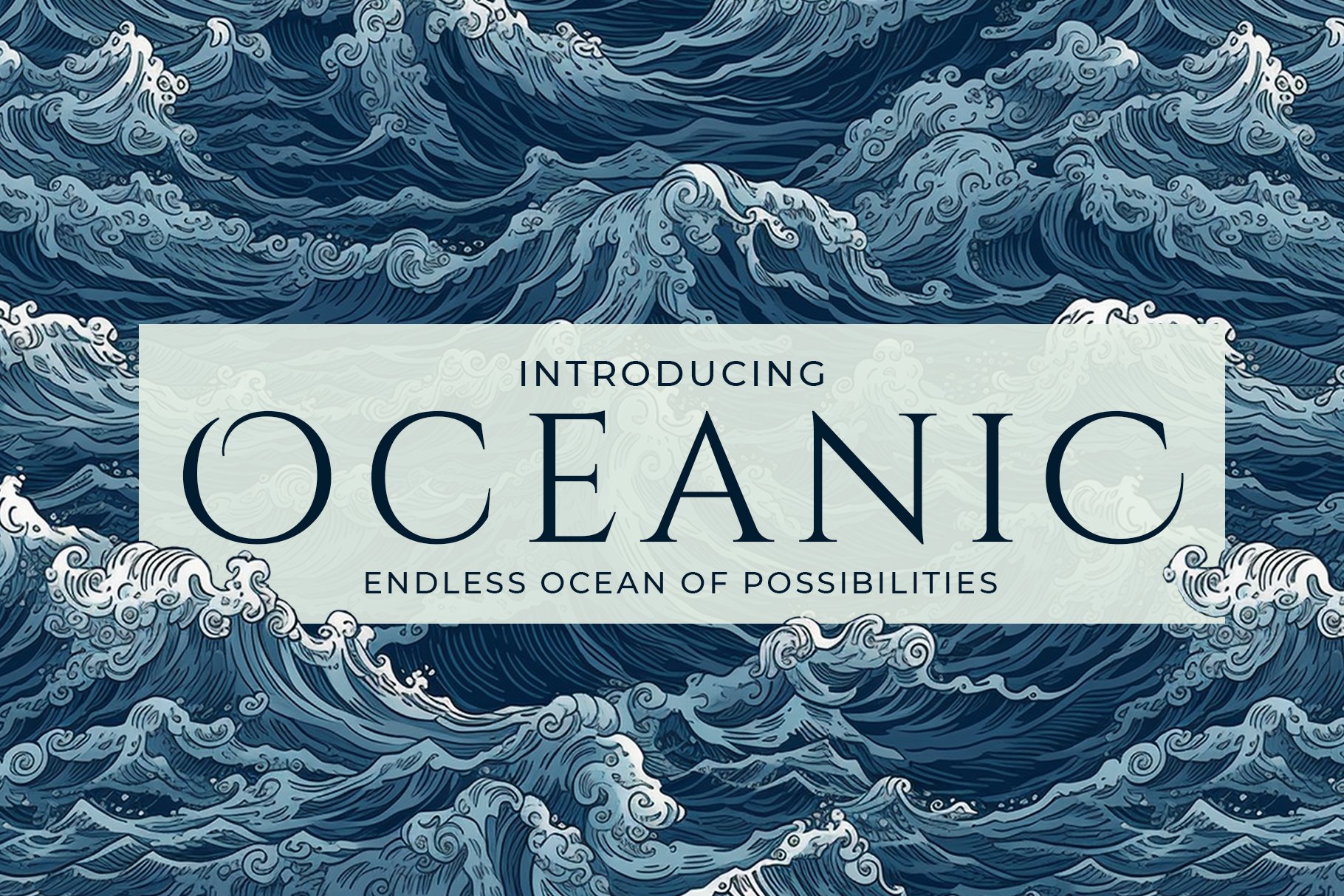The advertisement poster for "Oceanic" features a detailed, hand-drawn depiction of a vibrant and tumultuous ocean with blue waves capped with white froth and bubbles. The waves are dynamic, filled with curlicues and darker troughs, creating an impression of an angry, restless sea. Centered both horizontally and vertically against this backdrop is a prominent and clear message in block capital letters: "Introducing Oceanic" followed below by "Endless Ocean of Possibilities." The primary lettering "OCEANIC" is large and dark, either in black or a very dark blue, standing out against a lighter blue rectangular background that merges with the ocean waves at the bottom corners. The overall color palette is limited to three or four shades of blue and white, emphasizing simplicity and clarity while conveying the vast and powerful theme suggested by the text. This minimalistic yet striking design could suggest various ocean-related venues or services, such as an aquarium, a beach resort, a restaurant, or a hotel, though no further details are provided.